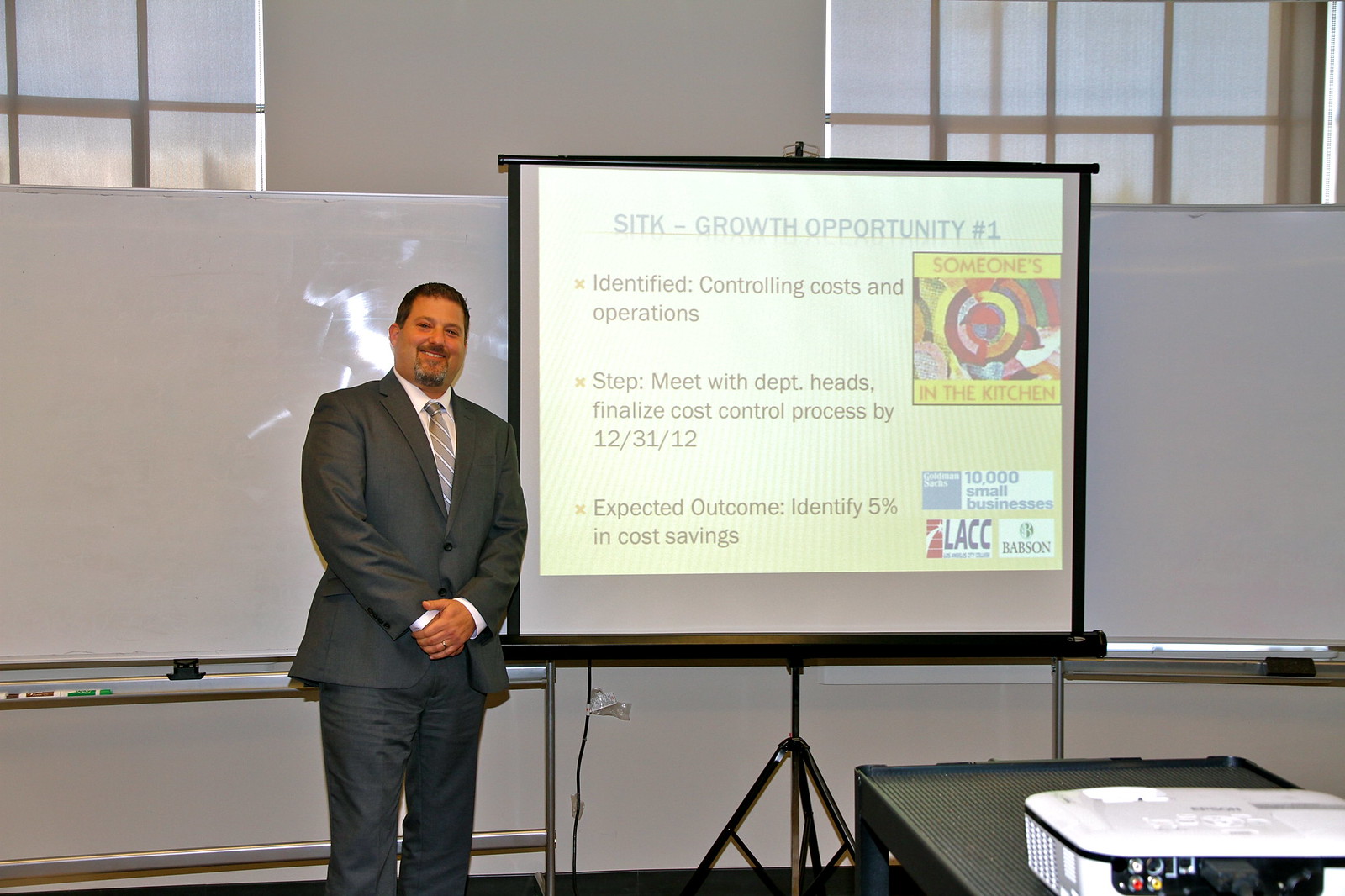The image captures a detailed view of a business presentation taking place in what appears to be a university classroom or professional setting. A white male with short dark hair, a goatee, and a mustache stands at the center, smiling at the camera while clasping his hands in front of him. He is dressed in a dark gray suit. Behind him, a projector displays a slide titled "SITK, Growth Opportunity Number One," detailing steps such as "Controlling cost and operation," "Meeting with department heads," "Finalizing cost control process by 12/31/12," and "Expected outcome: identifying 5% in cost savings." The man stands in front of a whiteboard positioned to his left. There is a table to the right of the image, holding a plastic bin or possibly another piece of equipment. The setting includes carpet flooring and appears to be indoors with natural daylight filtering through two windows located in the upper left and right corners of the room. The overall scene is vibrant, featuring a variety of colors including white, black, gray, silver, red, yellow, orange, pink, and purple.